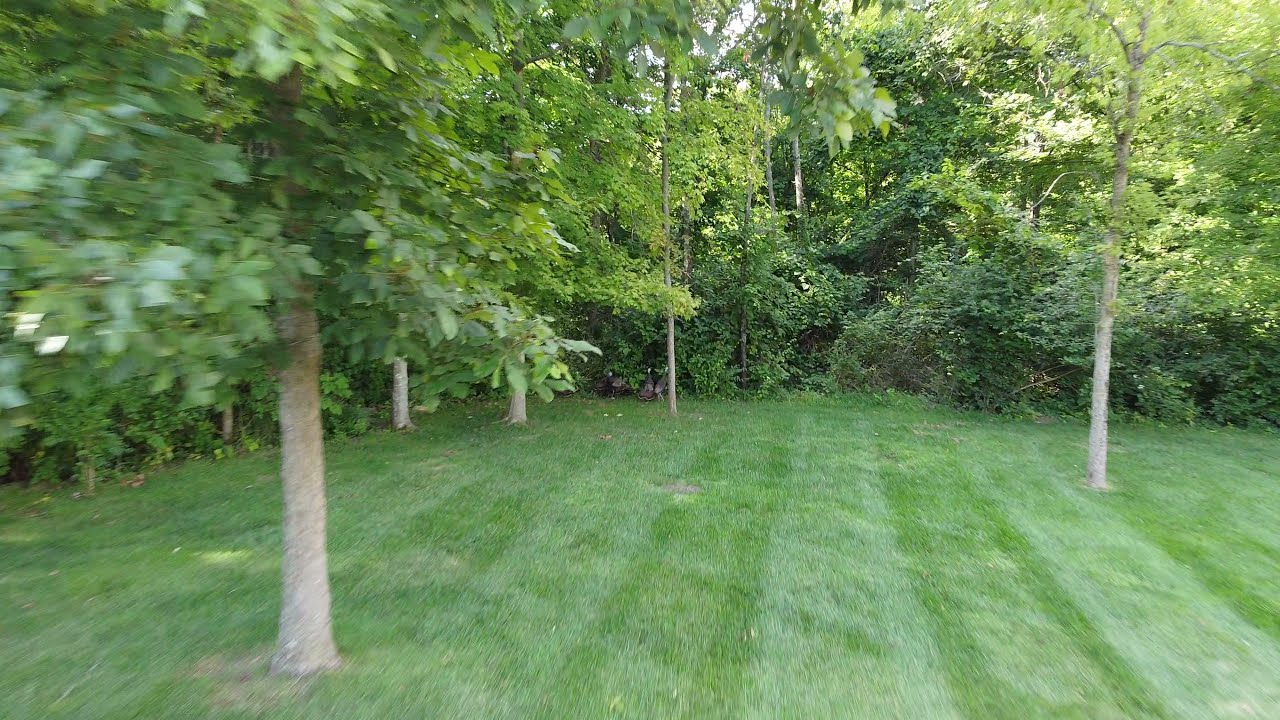This image showcases a meticulously maintained, freshly mowed grassy lawn area, likely part of someone’s backyard. The lawn displays distinct mowing stripes running vertically, alternating between darker and lighter shades of green. There are five trees positioned strategically around the lawn: one on the left-hand side near the bottom, two rising beyond it in parallel, a fourth tree to the right of the first pair, and a fifth tree situated towards the middle right of the image. 

The left side of the lawn is bordered by a dense arrangement of brush and bushes, which continues behind the trees at the far end, forming a natural barrier. This dense greenery extends into the background, where more tall trees stand, their lush green leaves hinting at a vibrant summer day. There is a hint of clear sky visible through the branches and leaves, enhancing the summery atmosphere. The image captures only the left and top boundaries of the lawn, leaving the extent on the right and bottom edges undefined. The well-maintained appearance and detailed vegetation suggest an inviting and serene outdoor space, likely part of a residential property.